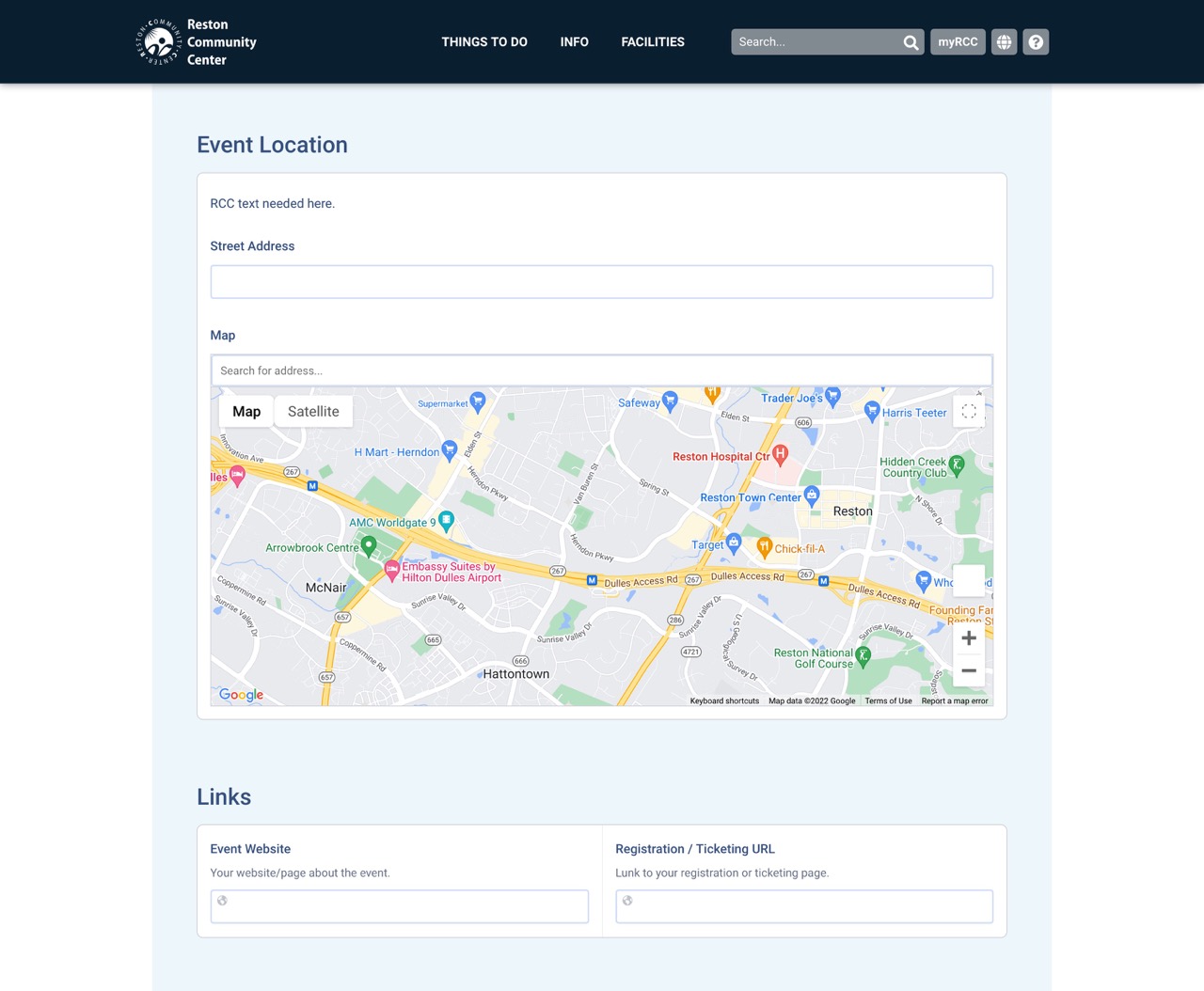This is a detailed screenshot of the Reston Community Center webpage. At the top left corner of the black header, "Reston Community Center" is prominently displayed alongside the organization's logo. The header features three navigational tabs labeled "Things to Do," "Info," and "Facilities," situated to the right of the center's name. Adjacent to these tabs is a search bar, followed by three functional buttons labeled "My RCC," along with a question mark icon and a globe icon.

The main content of the webpage has a clean, white background. Dominating this section is a heading titled "Event Locations," under which a meticulously organized chart is displayed. The first row of the chart indicates a placeholder text, “RCC text needed here,” followed by sections for a street address and a mapped area.

The map, situated prominently within the city of Reston, highlights the regions of Reston, Hattontown, and McNair. It also features a search address bar at the top for user convenience. Below the map is a section titled "Links," enclosed in a white box. This box contains two distinct areas: on the left, the label "Event Website" accompanied by a descriptive text, “Your website page about the event,” followed by a small text input bar. To the right, under "Registration," there’s a “Ticketing URL” label, also paired with a small text input bar.

This detailed caption captures both the layout and the specific elements present on the Reston Community Center webpage, providing a clear and comprehensive description.